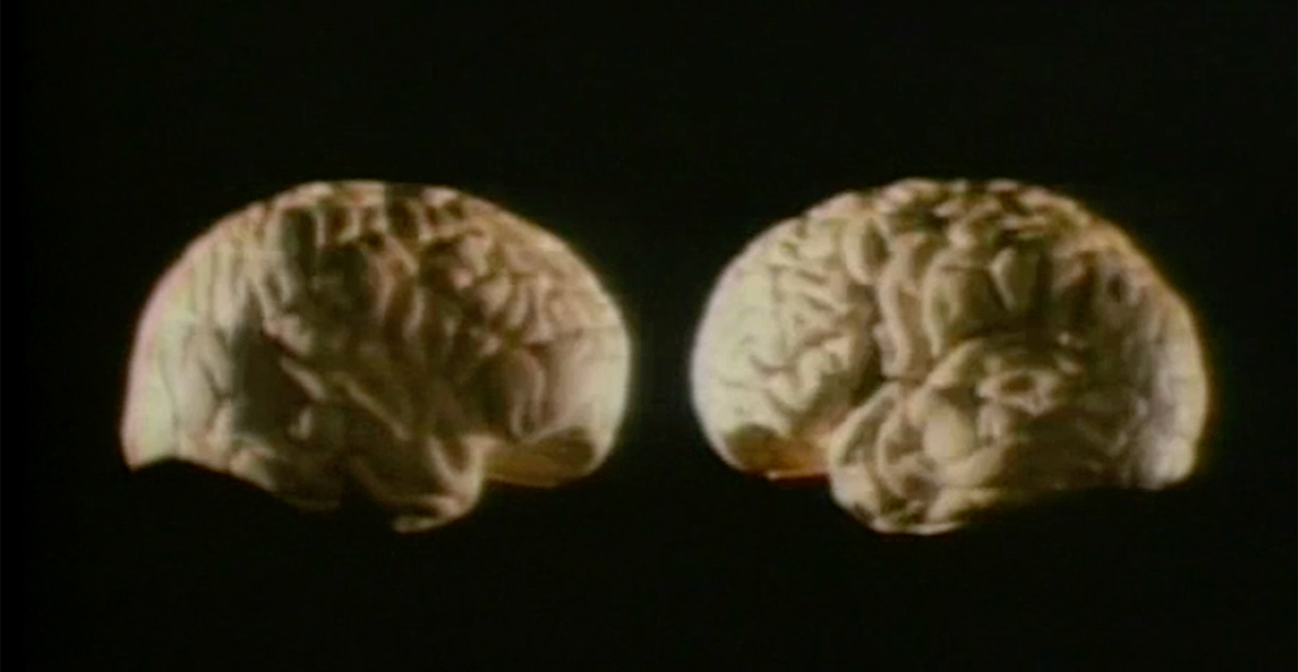This image depicts what appears to be two brain-like structures set against a completely black background. These structures, both resembling the shape and texture of human brains, display an off-white to pale yellow hue with darker shading in their cores. Positioned side by side, the structures exhibit the characteristic lumps and crevices associated with brain matter. Their coloration varies slightly between them; the left one has more distinct darker shades in the middle, whereas the right one is lighter overall. The image quality is somewhat blurred, suggesting it might be an older photo or a stylized artistic representation. The depiction suggests either two separate brains or a single brain showing both hemispheres set side by side.